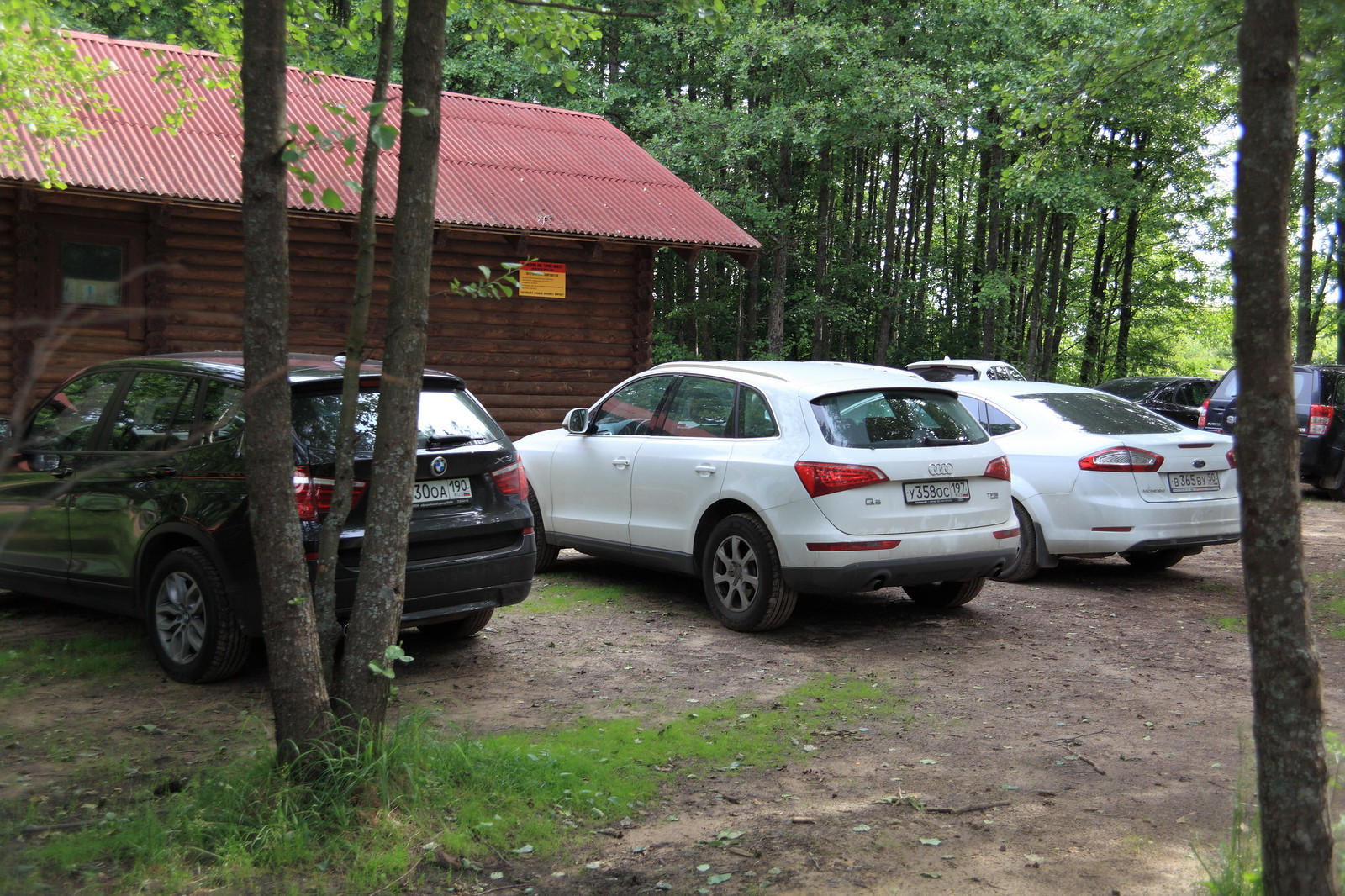In this detailed, real-life color photograph, a rural woodland setting unfolds with a log-sided cabin as the focal point. The cabin, characterized by its slanted corrugated maroon roof, occupies the mid-ground of the image and extends to the left border. Parked on bare dirt and mossy ground are three cars facing the cabin: a black BMW on the left, a white Audi in the center, and a potentially white Ford on the right. The backs of these cars are prominently visible. Thin tree trunks and mossy ground populate the foreground, and a yellow and red sign with black lettering adorns the cabin's exterior. Behind the cabin and these central cars, the background is a dense stand of young, tall trees with intermixed patches of sky and additional parked cars—two black and one white—peeking through the foliage. The scene captures a cloudy rural day devoid of people, with all elements crisply in focus.